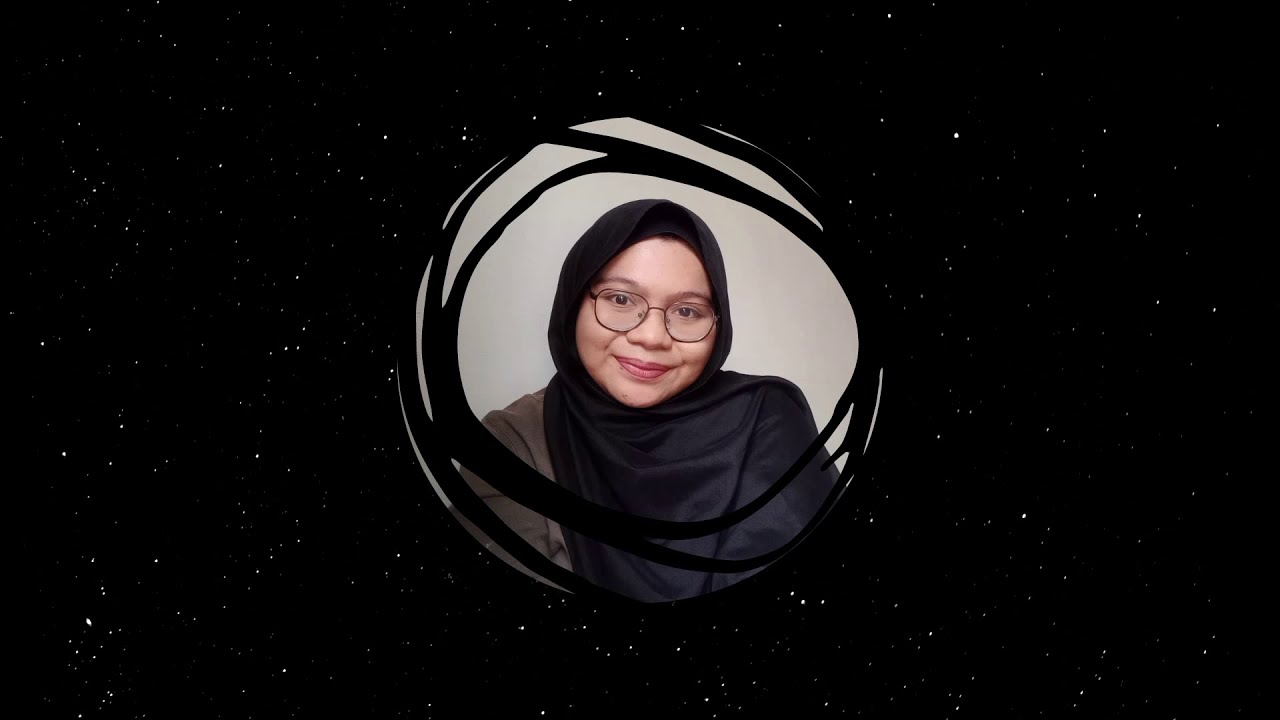The image captures a young woman, possibly of Muslim descent, against a primarily black background accentuated with tiny, star-like white dots. At the center is a light grey circle, overlaid with the woman's face. She wears a black headscarf that extends to her shoulders and down to her belly, which is where the picture cuts off. The headscarf closely frames her wide face, which features high cheekbones, a broad nose, and a wide smile, though she is not showing her teeth. Her big, wireframe glasses highlight her expressive eyes and normal-looking eyebrows. Surrounding the circumference of the grey circle are several random black circular lines, giving an artistic flair reminiscent of open circle swirls or branches. Her smile exudes warmth and openness, enhanced by her slightly tilted head, suggesting a receptive and approachable demeanor.